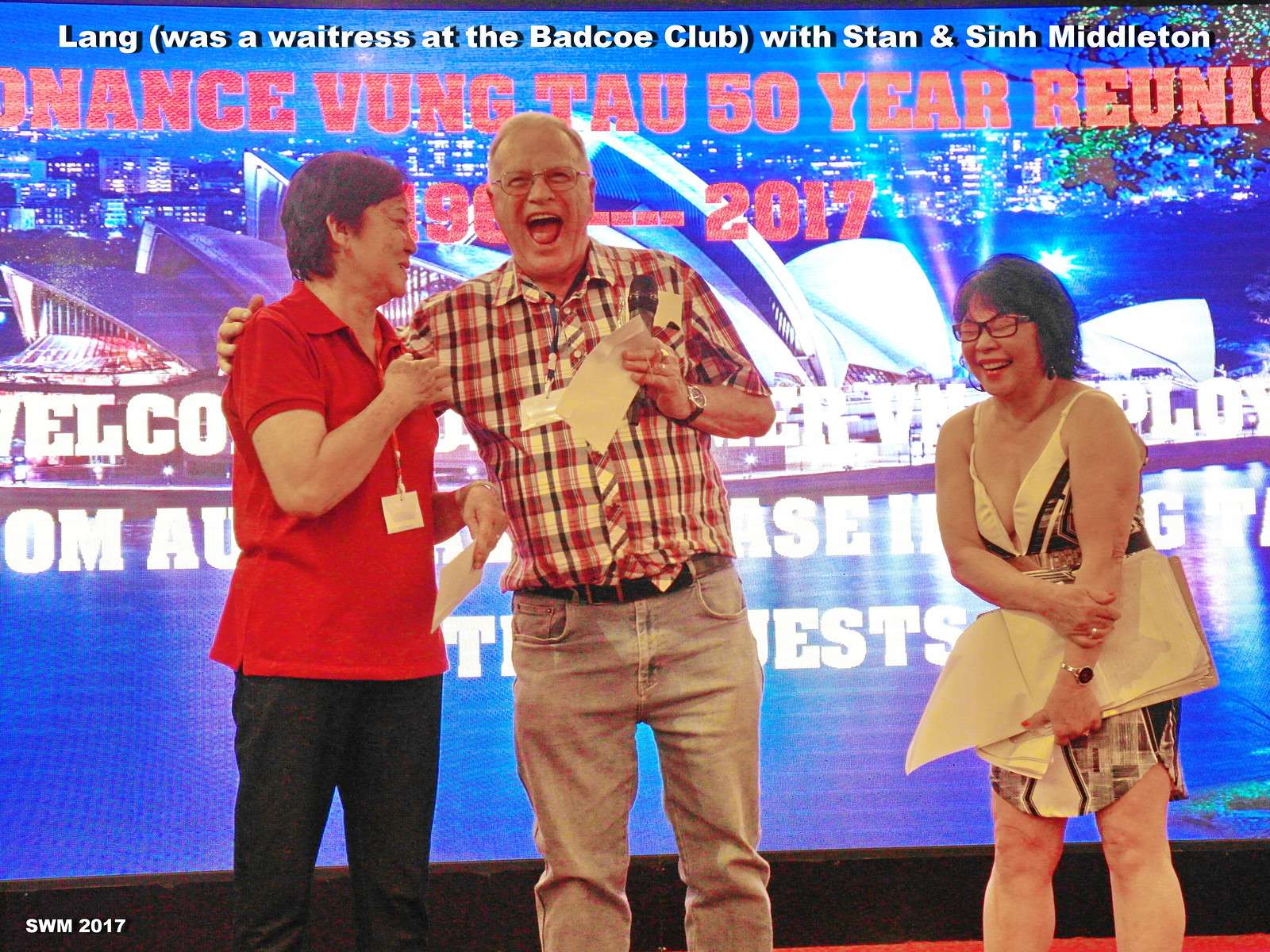On a well-lit stage, three individuals stand before a large screen showcasing a blue backdrop with a detailed cityscape and an inscription in white font. The screen prominently reads, "Lane was a waitress at the Badco Club with Stan and Sing Mendleton," and below it, although partially obscured, the text mentions the "Vung Tau 50 year reunion," spanning from "1960-something to 2017." On the left, a man of Asian descent, clad in a red shirt and black pants, carries an ID lanyard and directs his gaze towards the man in the center. This central figure, an older man with glasses, jovially clasps a microphone and a piece of paper in one hand while his other arm embraces the man on his right. He is dressed in a short-sleeved red, black, and white plaid shirt paired with blue jeans and a belt. To the right, a woman, also of Asian descent, sports a short, low-cut dress with thin straps, revealing her arms and legs. She wears dark, cat-eye glasses and holds several pieces of paper, laughing with her eyes shut. The backdrop hints at a reunion event, with a faintly visible image of the Sydney Opera House adding an element of international flair.